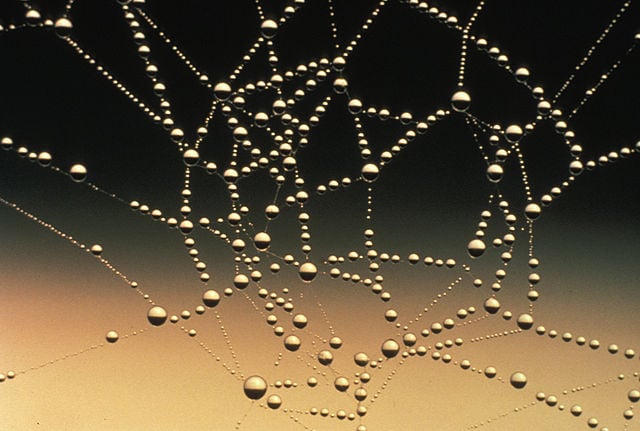The photograph captures an intricate spider web adorned with shimmering raindrops of various sizes. The web is primarily circular in design, composed of concentric circles. Within the web, some droplets form interesting shapes, including one that resembles a Star of David. The background exhibits a gradient of colors, beginning with a gold hue at the bottom, transitioning through shades of beige, rose, light gray, and darker gray, before finally becoming black at the top. This gradient causes the droplets to reflect different colors, with drops at the bottom appearing golden and those at the top appearing darker. The image is richly detailed with a multitude of water beads, some of which are large and prominent at the intersections of the web strands, while smaller droplets are scattered throughout. The contrasting background and the glossy appearance of the droplets give the web an almost magical, illuminated quality.